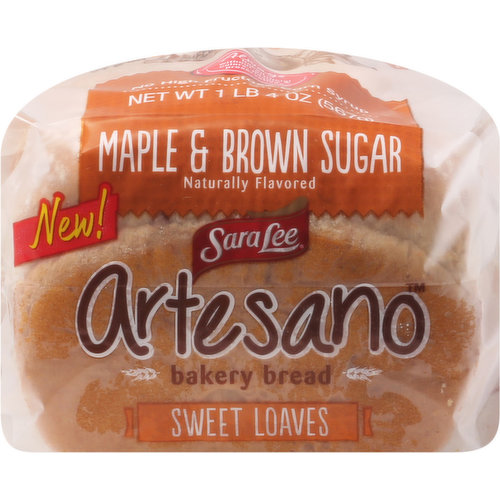The image depicts the back of a package of Artesano Bakery Bread by Sara Lee. The plastic packaging is see-through, allowing a glimpse of the brown-colored sweet loaves inside. The main brand "Artesano" is prominently displayed in a white font with a brown outline, while beneath it, "Bakery Bread" is written between two decorative leaves. Below this, on a reddish-brown rectangular ribbon, the product type "Sweet Loaves" is highlighted in white text. The package details include the net weight of 1 pound, 4 ounces (567 grams) and emphasize the naturally flavored maple and brown sugar concoction. The overall presentation suggests a delicious, new offering from the well-known bread maker, Sara Lee.